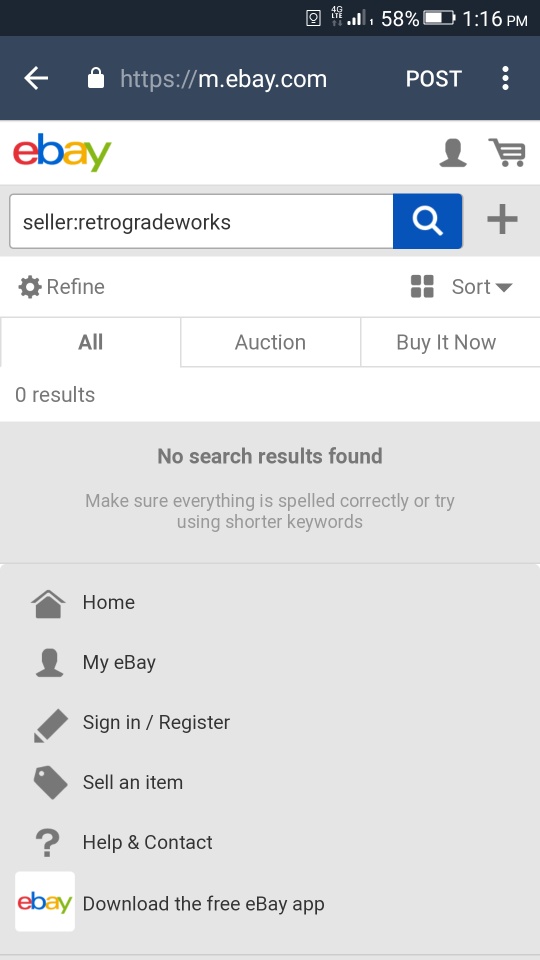The image is a detailed screenshot taken from a smartphone. The top border of the screen is black, displaying essential status indicators on the right side. The white font shows the time as 1:16 p.m., next to a battery icon indicating a 58% charge. The wireless signal strength is represented by four out of five bars illuminated.

Directly below this, the background shifts to a bluish-gray hue, featuring the web address "m.ebay.com" prominently. To the right of the address, white text displays the word "Post." Beneath this header, the main content of the eBay mobile website is visible against a white background. 

On the left side, the colorful eBay logo stands out with its distinctive lowercase letters: a red 'e,' blue 'b,' yellow 'a,' and green 'y.' In the search box next to the logo, the query "seller: retrograde works" is typed out. Below the search box, a light gray box spans the width of the screen, containing a darker gray font message that reads, "No search results found. Make sure everything is spelled correctly or try using shorter keywords."

Occupying the left side of the webpage, several menu items are listed vertically: "Home," "My eBay," "Sign in/Register," "Sell an Item," "Help & Contact," and "Download the free eBay app." Adjacent to the last menu item is a white square featuring the eBay logo once more.